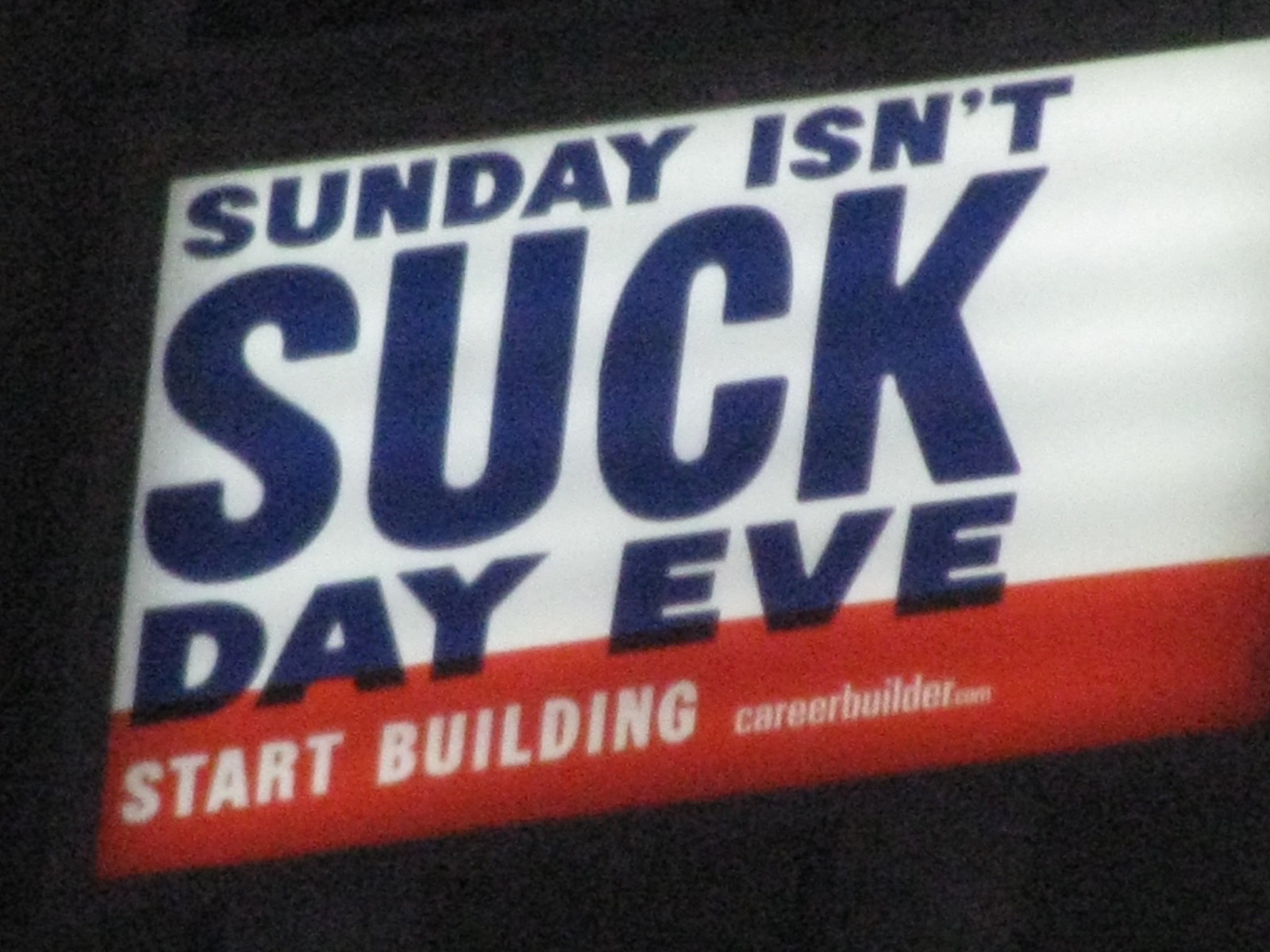This photograph captures a prominent light-up billboard set against a predominantly black, outdoor night sky. The rectangular billboard, brightly illuminated, dominates the center of the image, occupying over 90% of the frame. The upper portion of the billboard features a white background with the slogan "Sunday isn't suck day eve" displayed in big, bold, dark blue letters, with the word "suck" notably larger than the other words. Beneath this, a red background spans the width of the billboard, bearing the phrase "start building" in white text, with "careerbuilder.com" listed to the right in smaller white letters. The stark contrast between the brightly lit billboard and the dark, staticky surroundings enhances the visual impact of the advertisement.